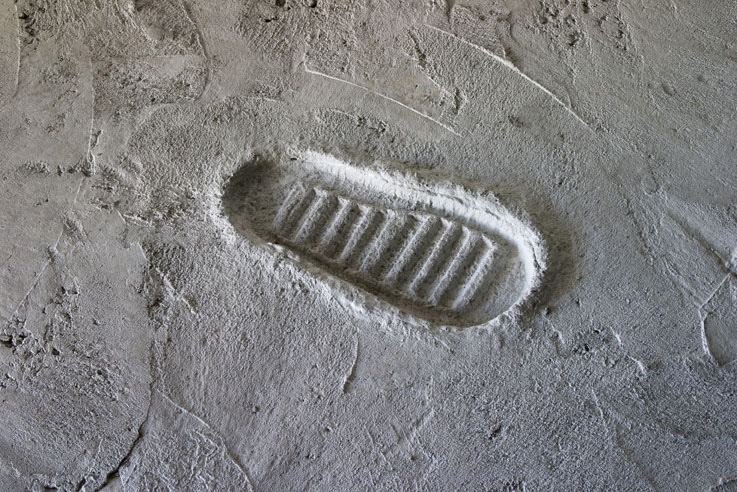In this detailed photograph, we see a single, prominently imprinted footprint on a light gray sandy surface. The surface, while mostly flat, is marked with various scratches, pits, cracks, and irregular shapes, lending it a rugged, textured appearance. At the center of the image lies a deep, well-defined boot print, characterized by its oval shape that's thicker at one end. The boot sole that created this impression was designed with nine notable ridges, and these have been impressively transferred to the sand. The footprint, left by a large boot, is surrounded by a rectangular frame of the image, capturing the granularity of the surface and the precise details of the boot’s sole pattern.